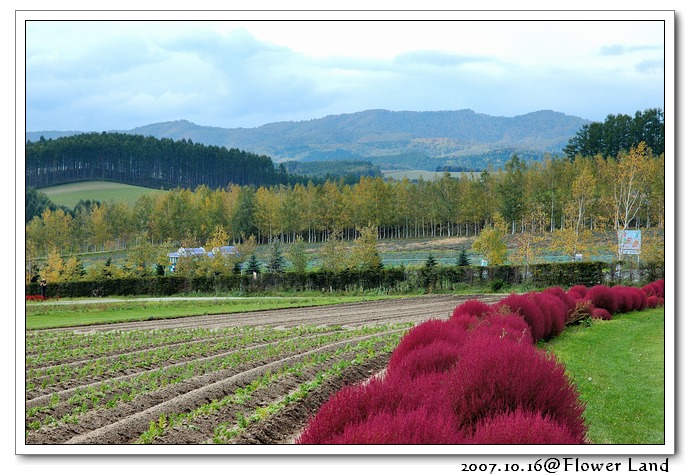This photograph, bordered with a thin black-white-black frame, is dated 2007.10.16 at Flowerland. The outdoor landscape from front to back begins with neatly arranged rows of plants in heaped mounds, curving from left to right towards the mid-horizon. To the right of these rows, a vibrant border of purplish-red, spiky flowering shrubs transitions into a grassy area. Central to the image are small deciduous shrubs and trees, extending towards the backdrop. Further into the scene, a house or greenhouse is visible, accompanied by additional rows of plants behind it. The middle ground expands into a meadow with a mix of deciduous and coniferous trees, all set against the backdrop of bluish foothills and a thick cloudy sky, shaded in hues of white and gray. The detailed landscape likely belongs to a plant nursery or arboretum, capturing a serene countryside ambiance.